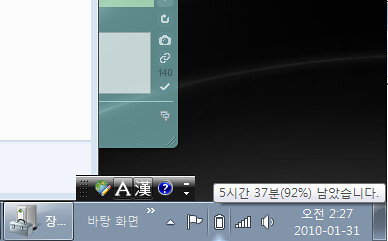The image appears to be a screenshot of a digital screen with a predominantly dark background, likely from a computer or a mobile device. On the left side, there is a visible portion of a light blue smartphone or app interface. This section of the screen features several icons including a refresh icon, a camera, two chain links, the number 140, a checkmark, and two screens. Below these icons are additional symbols: a pencil on a globe, a letter 'A', an Asian character, and a question mark. Underneath this is a white box displaying the numbers 5, 37, and 92% along with more Asian characters.

At the bottom left-hand corner, there's a toolbox icon followed by another box with Asian characters and a flag icon. Additional icons in this area indicate battery level, volume, and a microphone, with the numbers 2, 27, and the date 2010-01-31 also displayed. To the right of the light blue section is a white rectangle bordered in blue, followed by a gray-rounded rectangular section and another gray box. The rest of the screen, extending towards the right, is mostly black with a streak of gray running horizontally. The display includes several colored rectangular sections scattered within this black area, creating a fragmented mosaic of information against the dark background.